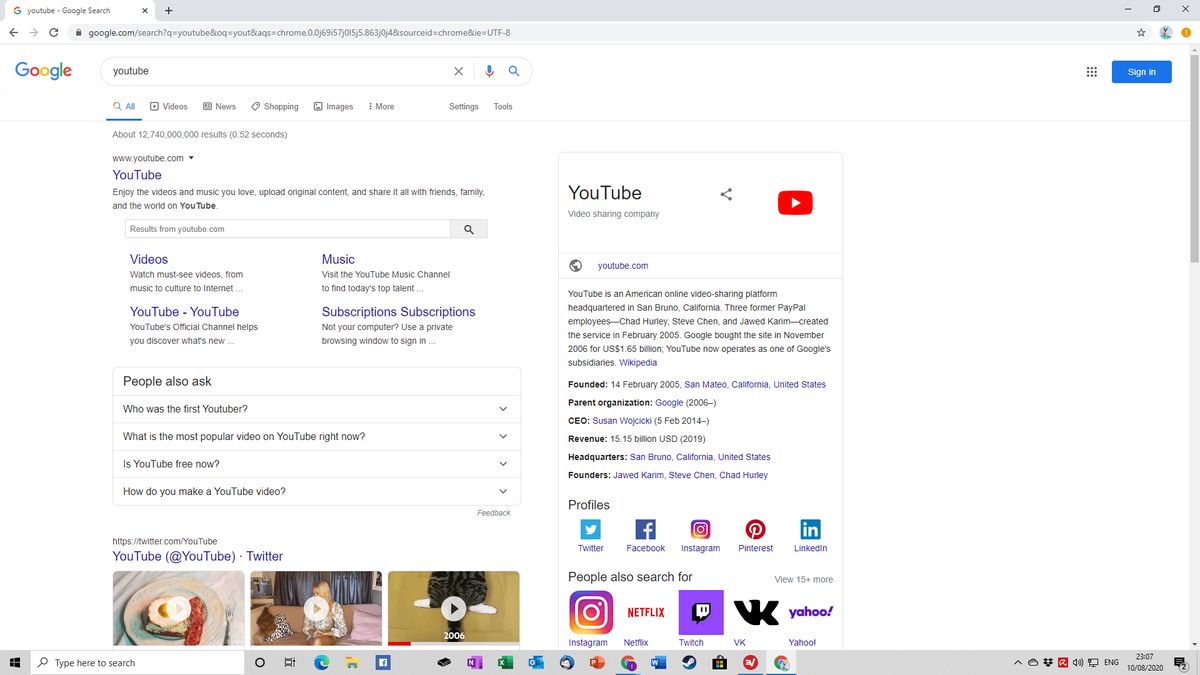The image depicts a computer screen with the search term "YouTube" entered into a web browser, displaying the top result as YouTube.com. The user's taskbar, indicative of a Windows operating system, is visible along the bottom, featuring a variety of icons including Steam, Chrome, Microsoft Office suite applications, Microsoft Edge, and File Explorer. 

The search result for YouTube is expanded, presenting quick access links to various subcategories such as videos, music, and subscriptions. On the right side of the screen, there is a side pane offering quick links to related content, including a Wikipedia entry for YouTube, social media profiles, and additional resources.

Further down, the "People also ask" section provides commonly queried information such as "Who was the first YouTuber?", "What is the most popular video on YouTube right now?", "Is YouTube free now?", and "How do you make a YouTube video?". Scrolling down more, you can see embedded video previews from the YouTube Twitter account, one featuring a breakfast plate and another showcasing a woman sewing against a white background.